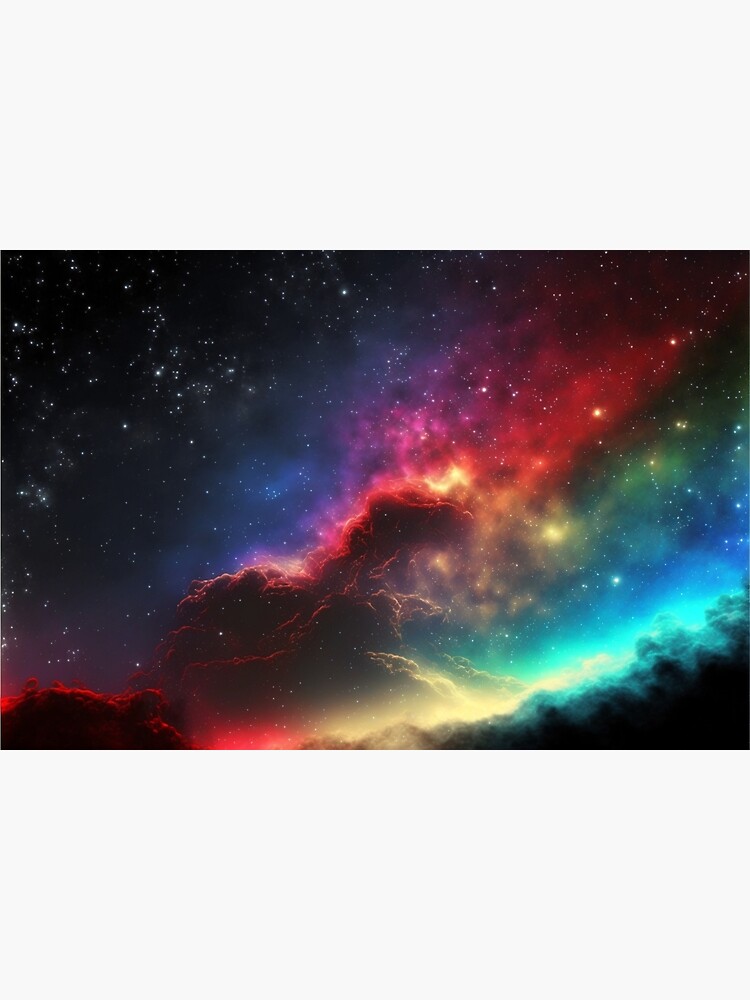The image presents a digitally-rendered or computer-edited depiction of a cosmic scene, blending both artistic elements and realistic details. The top left corner begins with a deep black sky peppered with small white stars. As the eye moves diagonally towards the bottom right, the sky transitions smoothly from black to a rich blue, and then to a vibrant purple. This gradation continues into a striking red and yellow section, where the colors are interspersed with ethereal cloud formations that primarily retain the red hue before blending into yellow. In the center of the image, a bright star is surrounded by pink, red, and blue clouds, suggesting a stellar nursery or a nebular region. Moving further down, the image transitions into bands of green and light blue, dotted with white and yellow lights reminiscent of distant stars. The color palette finally shifts back into a dark, almost black area, with additional cloud formations tinged with bluish hues. Overall, the image captures the essence of a galaxy or nebula, with all the colors of the rainbow presented in smooth and harmonious transitions, enriched with star clusters and multicolored clouds, lending a surreal yet strikingly beautiful quality to the cosmic landscape.